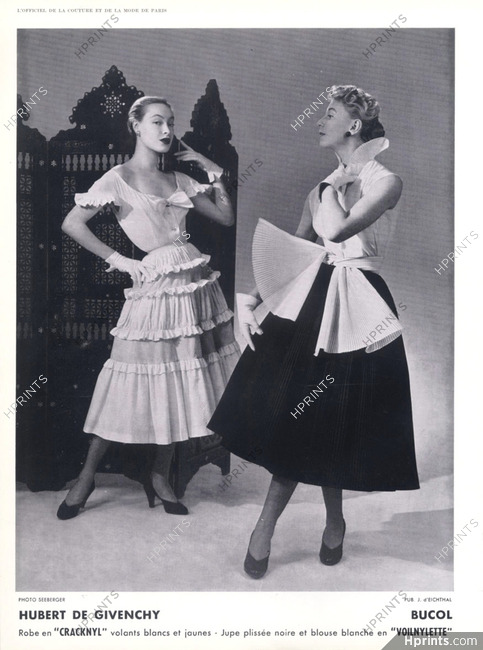The black and white image displays two women, likely models, against a light-colored background with a dark, ornate wooden room divider behind the woman on the left. Both women are dressed elegantly. The woman on the left, standing slightly angled to the right, is wearing a white dress with four tiers of ruffles from the waist down and short sleeves. She completes her look with black heels and gloves, with her left hand near her cheek and right hand on her hip. 

The woman on the right, facing back towards the first woman, is wearing a sleeveless white top with a high collar and a very ornate white bow at the waist, paired with an A-line black skirt, also around T-length. She has black shoes, short blonde hair, white gloves, her left arm up by her neck, and her right hand resting by her side.

Across the image, from the bottom left going up to the right at an angle, are the words "HP Prince." In the bottom left corner, there's small black text reading "Hubert D. Givenchy," followed by more black print extending across the entire bottom of the picture. The bottom right corner features "BUCOL" in black letters, and beneath this area is a small gray bar displaying "HPPrince.com."